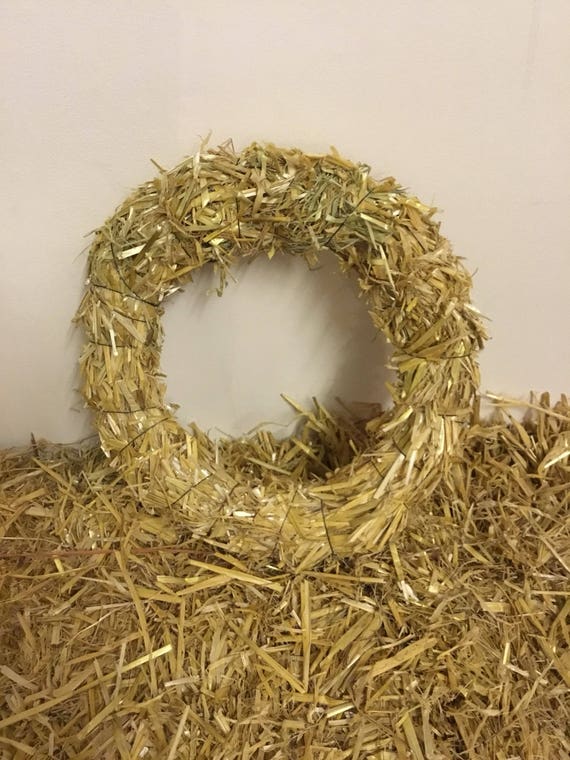The image depicts a wreath crafted from golden-yellow and tan hay, meticulously bound together using black string and twine to maintain its circular shape. This handmade wreath is positioned atop a large, scattered pile of loose hay, giving the appearance of a rustic bed of straw perhaps intended for animals. The entire arrangement is set against a plain white wall, devoid of any text or human presence, creating a simple yet striking composition.